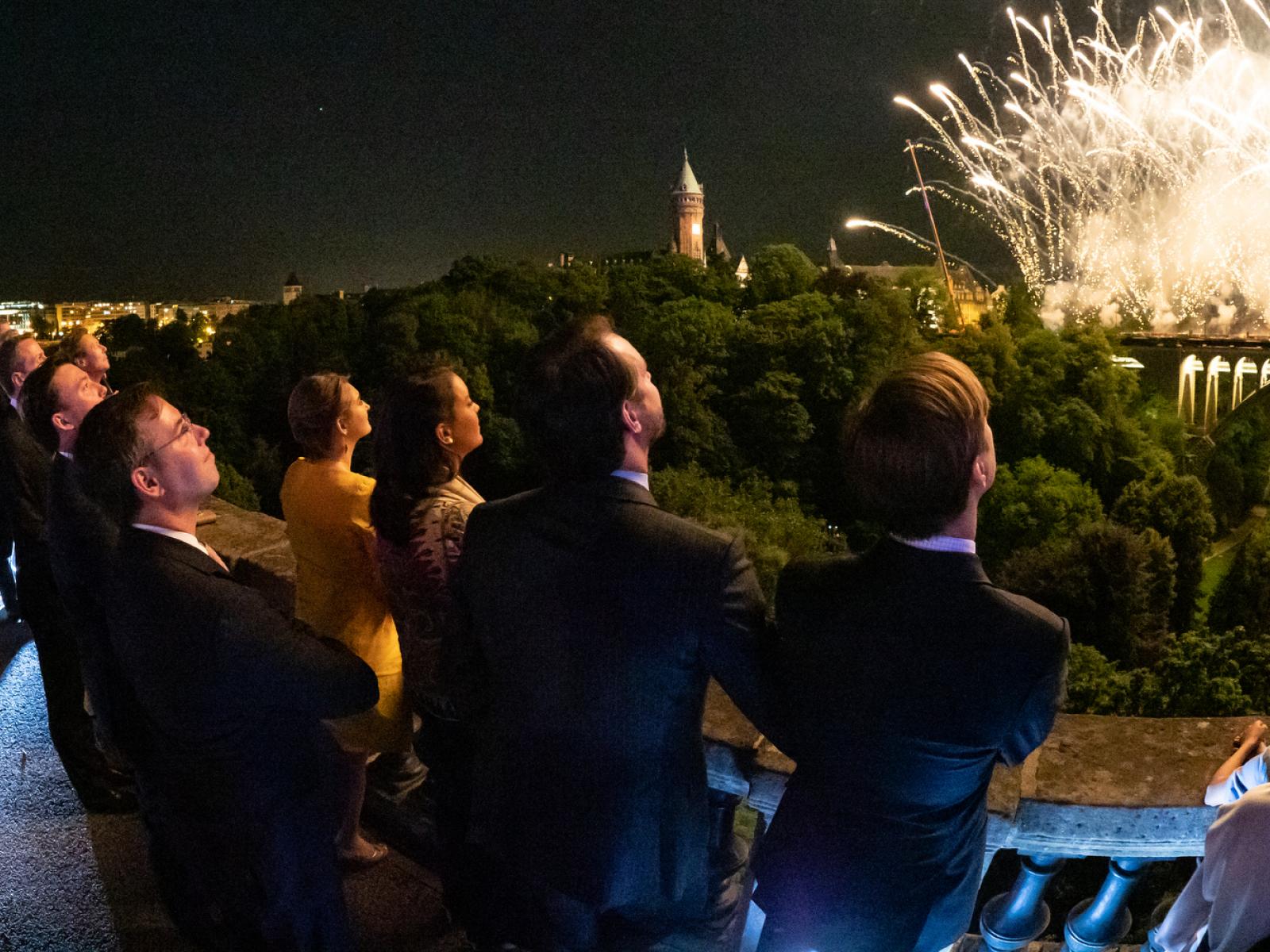In this nighttime photograph, eight people, comprising six men and two women, stand watching a spectacular fireworks display with awe. The sky is a deep black, illuminated by big, yellow-white fireworks shooting upwards, predominantly on the right side of the image. The grandeur of the event is highlighted by the participants' attire—men dressed smartly in black suits and women wearing elegant dresses adorned with regal jewelry. The setting seems formal, possibly involving politicians or another high-status gathering. In the background, a large tower is faintly visible, and dense clusters of trees frame the fireworks. The spectators are elevated, suggested by the railing visible at the bottom left. Although you mostly see the backs of their heads, a Caucasian man in the bottom left is distinguishable, wearing glasses and a suit, his profile partially visible as he looks on. Their posed, synchronized gazes towards the fireworks add an almost staged quality to the ambiance.